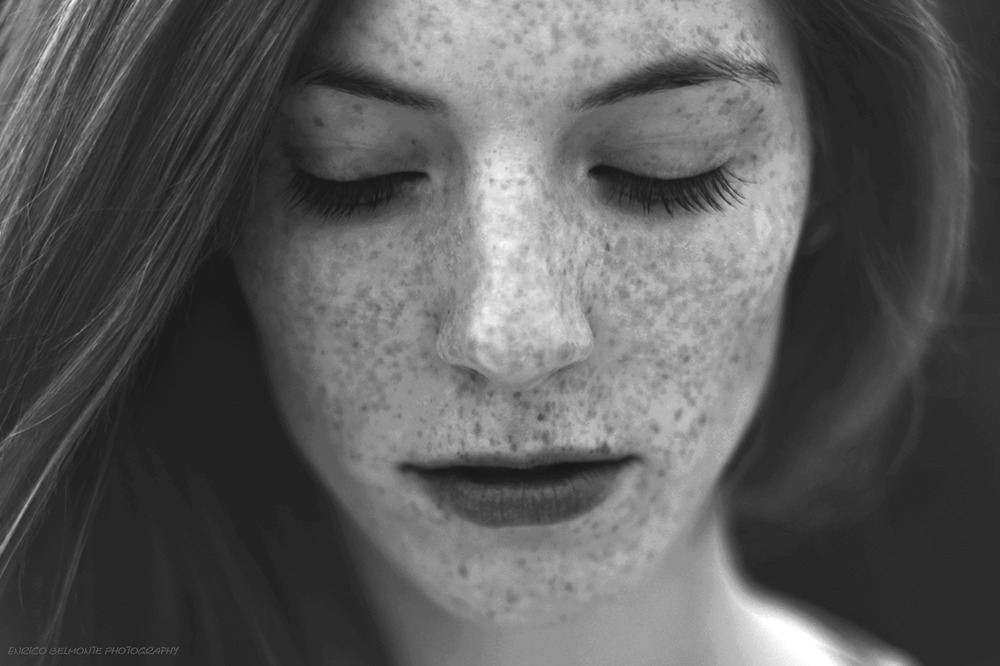This is a black-and-white, close-up photograph of a young woman, likely in her late teens or early twenties. The artistic composition of the image focuses predominantly on her face in an effort to evoke deep emotion and introspection. Her head is slightly tilted downward with her eyes closed, giving her a contemplative appearance. She has long, dark straight hair that falls smoothly over her left shoulder, and her face is adorned with numerous brown freckles that stand out against her pale complexion. Her dark eyebrows and exceptionally long black eyelashes frame her closed eyes. The photograph cuts off just below her chin and extends upwards halfway through her upper forehead, with part of her forehead going off-screen. The background is dark, enhancing the focus on her facial features. Her lips appear darker in color, and she seems to be wearing little to no makeup. The blurred areas around her shoulders and hair suggest a deliberate focus on her emotional expression.